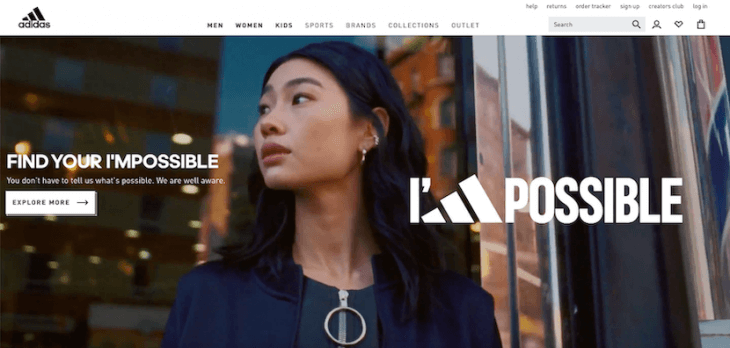In the image, there's a striking advertisement featuring a woman dressed in a stylish blue jacket paired with a green shirt. The jacket prominently displays the Adidas logo. A bold, empowering message overlays the image, stating, "I'm possible. You don't have to tell us what's possible; we are all aware." Below this message is a white rectangle with the call-to-action, "Explore More."

The top left corner of the image features the Adidas logo along with navigable categories including "Men," "Women," "Kids," "Sports," "Brands," "Collections," and "Outlet," with the categories "Men," "Women," and "Kids" emphasized in bold. At the very top of the image, additional navigation options are presented, such as "Help," "Return/Returns," "Water Tracker," "Sign Up," "Creators Club," and "Login." The interface also includes a search bar accompanied by profile, heart, and shopping bag icons, providing a seamless shopping experience for viewers.